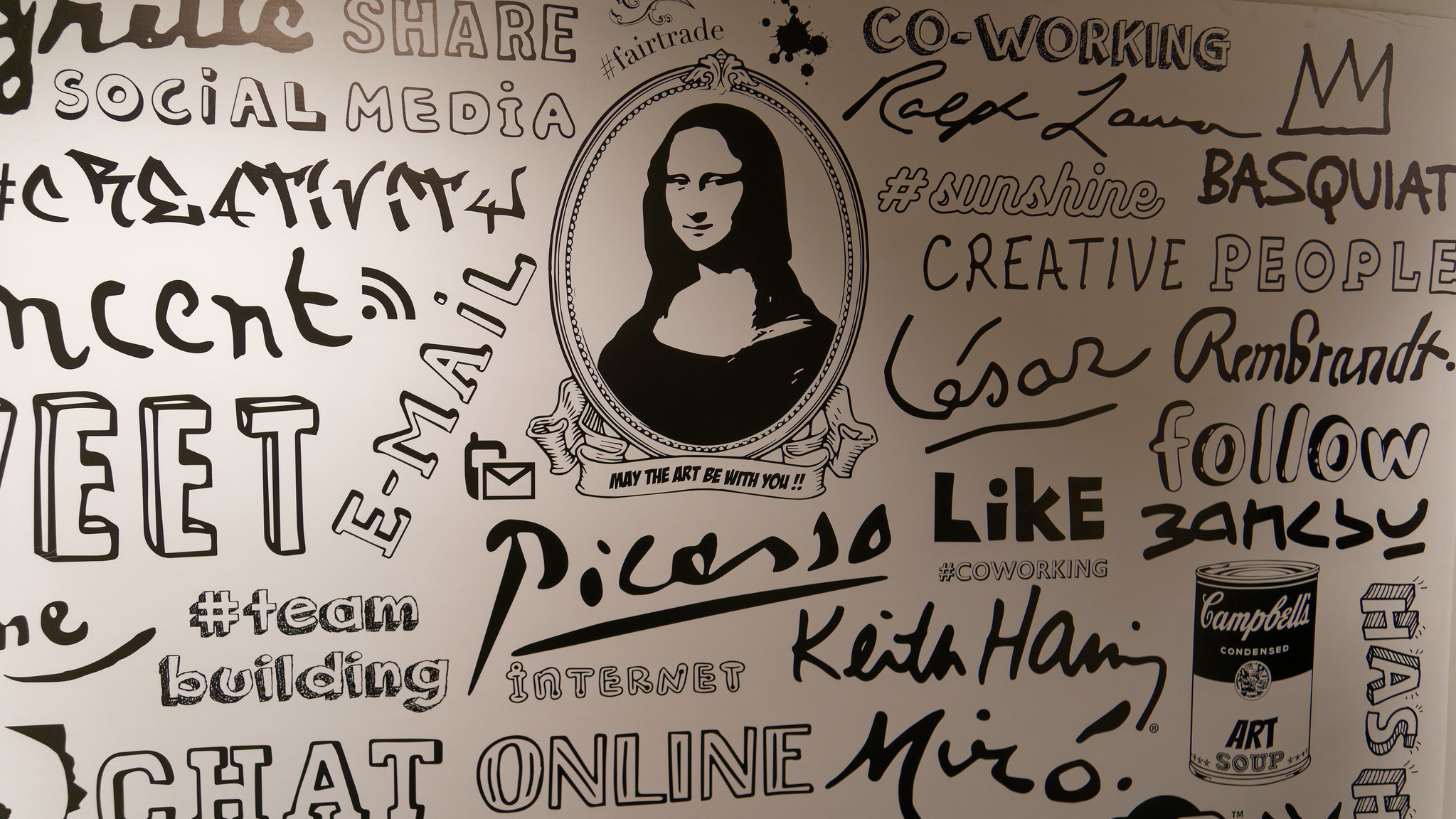The image features a wall designed as an artistic collage in shades of black, white, and gray. The focal point at the center is a black and white depiction of the Mona Lisa, framed in a quintessential English portrait style, with the phrase "May the art be with you" inscribed beneath it. Surrounding the central image, the wall is filled with various words and phrases in different fonts, such as "social media," "share," "email," "hashtag," "team building," "chat online," "internet," "co-working," "Picasso," "Basquiat," "Rembrandt," "follow," "creative people," "sunshine," and "like." On the bottom right corner, there is a drawing labeled “Campbell's Condensed Art Soup.” This creative setup likely decorates a wall in a shared co-working space, celebrating both artistic and modern digital culture elements.